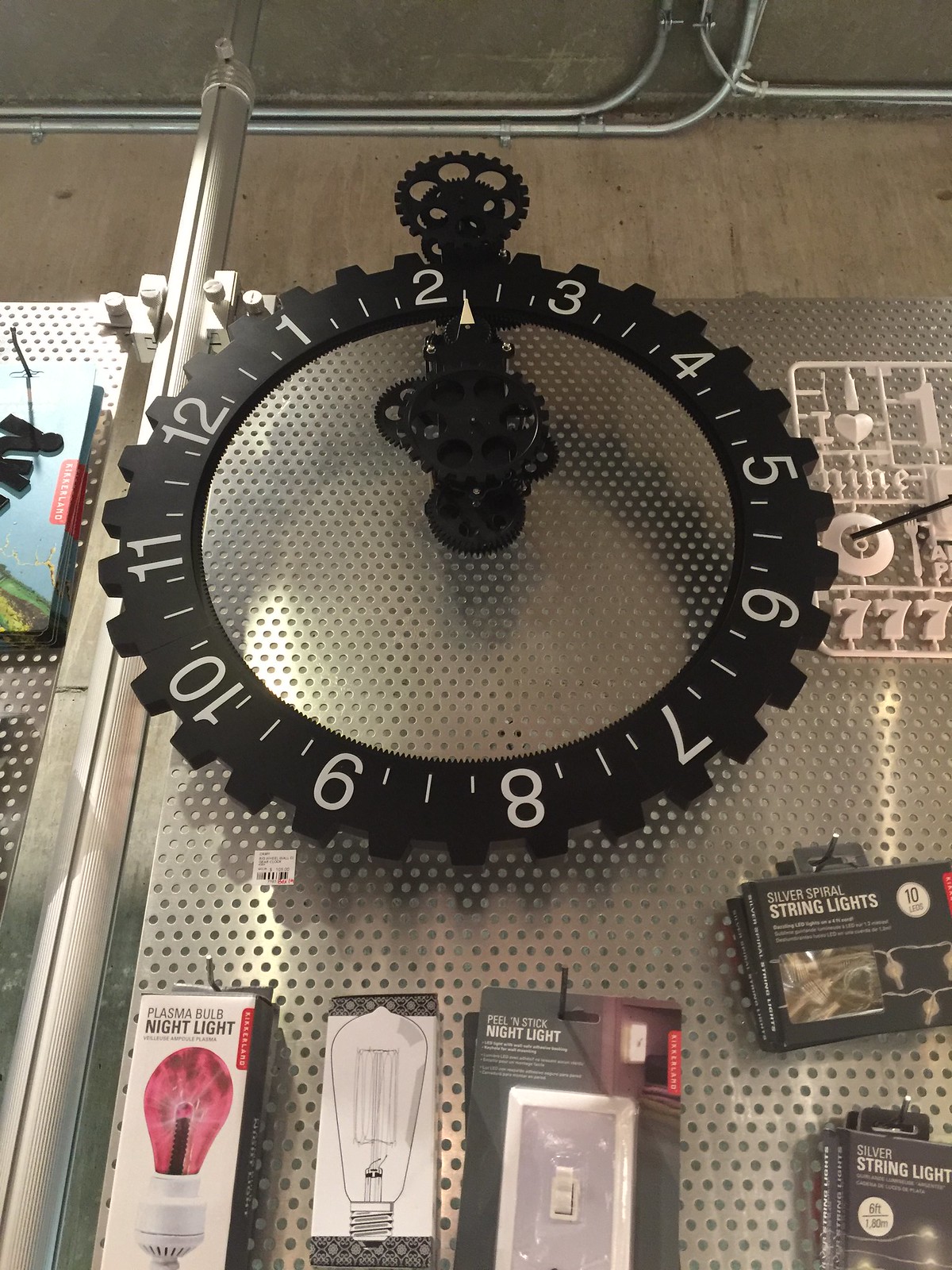The image depicts a uniquely designed wall clock prominently displayed in what appears to be a store setting. The clock itself is crafted to resemble a large, black gear, with intricate gear-like structures also integrated into the clock's design. The face of the clock features a white-silver interior adorned with numerous small dots, adding texture and detail. Above the clock face, additional black gears serve as decorative elements, enhancing the mechanical theme. Both the minute and hour hands are composed of clusters of smaller gears, reinforcing the industrial aesthetic. The clock is mounted on a silver backdrop, which appears to be part of a device or stand used for display purposes. Surrounding the clock, various store fixtures such as lights, bulbs, and switches are visible, indicating that the clock is available for purchase in a retail environment. The wall behind the display is made of gray concrete, providing a neutral background that accentuates the clock's striking design.